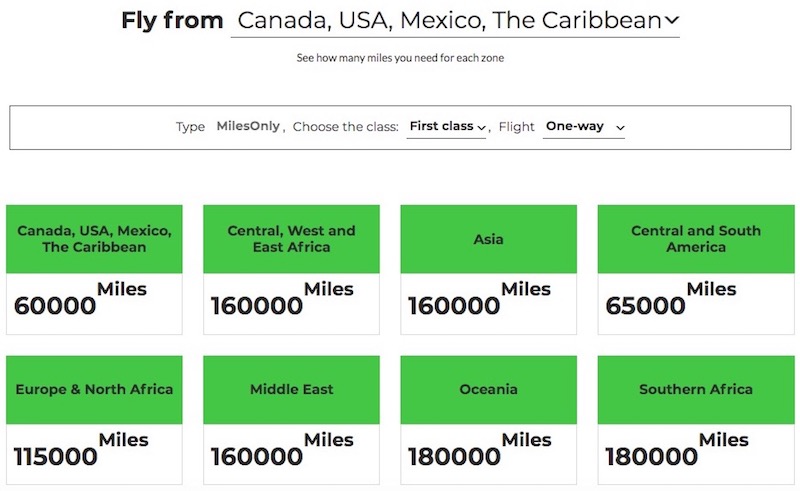**Caption for Image:**

This image is a screenshot from a website with a white background, featuring details about flight mile requirements for various global destinations. At the top, there is a section with black text listing "Fly from Canada, USA, Mexico, the Caribbean." Directly below is a black bar with a dropdown arrow, inviting users to "See how many miles you need for each zone." 

Further down, there's a black-outlined rectangle that contains options for inputting miles, selecting flight class (First Class from a dropdown menu), and choosing between a one-way or round-trip flight (dropdown menu options).

Below this input section are two rows of information boxes. The top row is green, and the bottom row is white, organized into four categories each:

1. Canada, USA, Mexico, the Caribbean: 60,000 miles
2. Central, West and East Africa: 160,000 miles
3. Asia: 160,000 miles
4. Central and South America: 6,500 miles
5. Europe and North Africa: 115,000 miles
6. Middle East: 160,000 miles
7. Oceania: 180,000 miles
8. Southern Africa: 180,000 miles

The image seems designed to inform the user of the required miles for flights to specific regions.